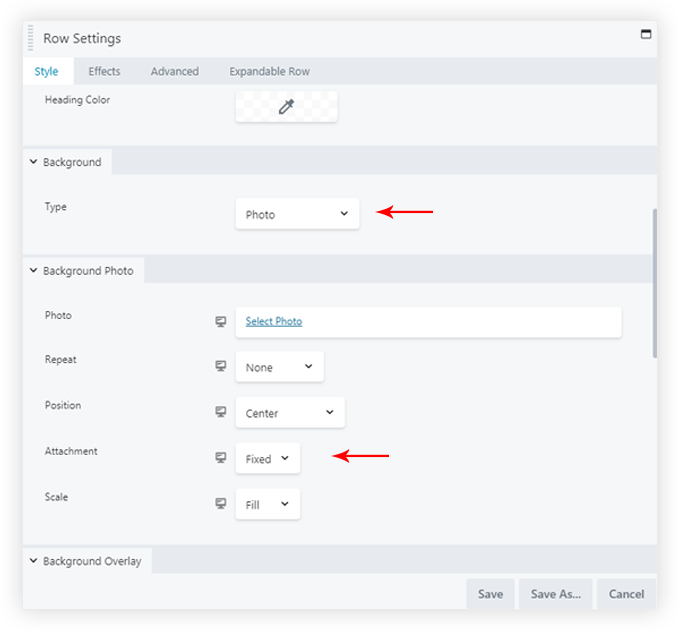This screenshot captures a website page dedicated to adjusting various settings. At the top of the page, the heading "Row Settings" is prominently displayed. Below the heading, a horizontal gray bar features four option tabs: "Style" (highlighted in blue to indicate it is currently selected), "Effects," "Advanced," and "Expandable Row."

Under the "Style" tab, the first adjustable setting is for the heading color. A gray and white checkerboard pattern with an eyedropper icon is visible, allowing users to select specific heading colors.

The next section focuses on the background settings. The first subcategory here is "Type," which includes a dropdown menu currently set to "Photo," indicated by a red arrow pointing to the selection. The subsequent subcategory is "Background Photo," which is itself divided into five further categories, each with a corresponding white selection bar to the right:

1. **Photo:** Displays "Select Photo" in blue and underlined within the white bar.
2. **Repeat:** A dropdown menu with "None" currently selected.
3. **Position:** A dropdown menu with "Center" selected.
4. **Attachment:** A dropdown menu with "Fixed" selected, indicated by another red arrow.
5. **Scale:** A dropdown menu with "Fill" selected.

Following the "Background Photo" section, there is a category labeled "Background Overlay," although its subcategories are not visible in the screenshot.

In the lower right corner of the page, navigation buttons are provided for saving, saving as a different file, or canceling the changes made. This layout ensures that users can easily modify and save settings efficiently.